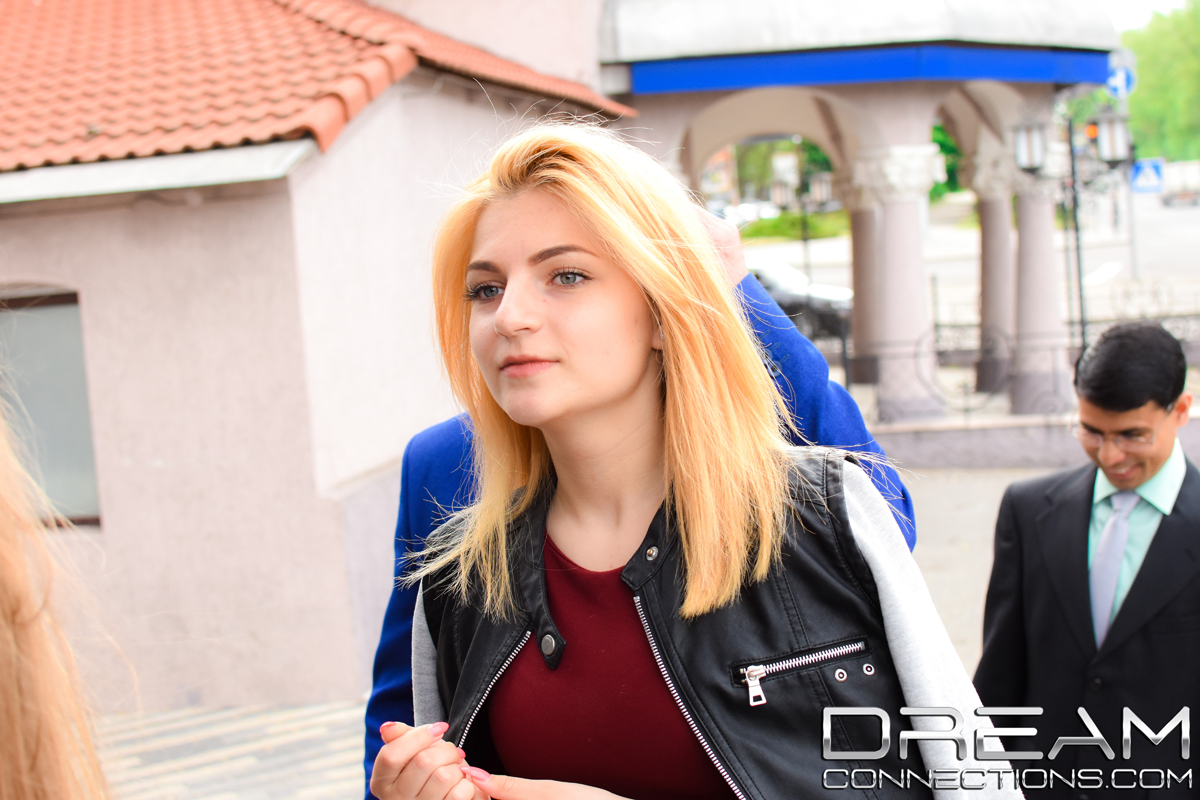In this outdoor daytime professional photograph, a young woman is the central focus, her figure sharply detailed against a bright, vivid backdrop. She has medium blonde hair and piercing blue eyes, with her gaze directed slightly to the left. The young lady is dressed in a red shirt with a black and white leather jacket draped over her shoulders, her manicured fingernails gently touching each other. Behind her, partially obscured and clad in a blue garment, stands an unseen individual. Further back to the right, a smiling man in a dark suit coat, mint green shirt, light tie, and glasses, looks down. The background reveals a stucco building with a red tiled roof, and another structure with blue detailing that leads into a street scene, complete with blurry street lamps and a few trees. The polished chrome silver watermark "DreamConnections.com" is distinctly visible in the lower right-hand corner.